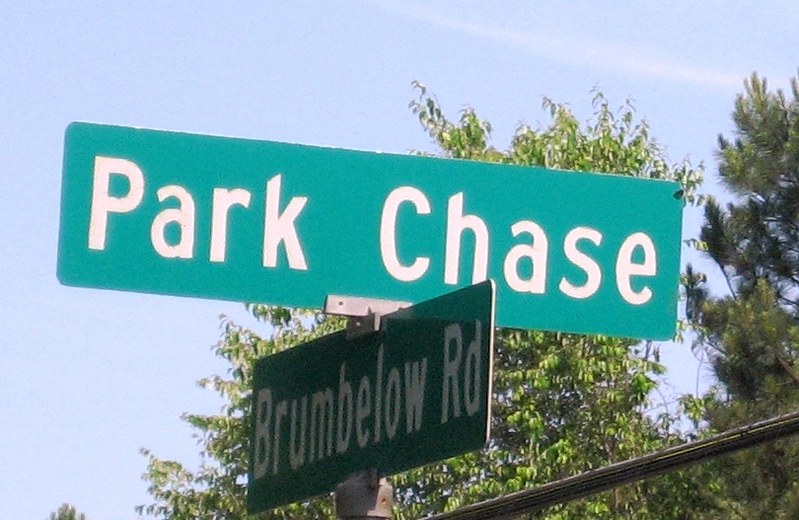This rectangular image, oriented horizontally, captures a clear, sunny afternoon at an intersection marked by two street signs. The scene is characterized by lush, green trees in full bloom, indicating a spring or summer day, against a backdrop of a vibrant blue sky adorned with a few wispy clouds. 

Prominently displayed in the photo are two green street signs with white lettering. The top sign, reading "Park Chase," extends from left to right. Slightly below it, a perpendicular sign labeled "Brumbelow Road" (spelled B-R-U-M-B-E-L-O-W, followed by "R-D") stretches diagonally from the bottom left to the upper right. Both signs are secured by silver metal pieces, with a rounded attachment device at the base of the Brumbelow Road sign, securing them together and to a pole that extends from the bottom center of the image toward the right.

A cable is faintly visible at the bottom, leading towards the right. The intersection scene is neatly framed by the contrasting shades of the two trees: one with lime green leaves and the other with darker green foliage, providing a natural canopy that enhances the serene and picturesque quality of the photograph.